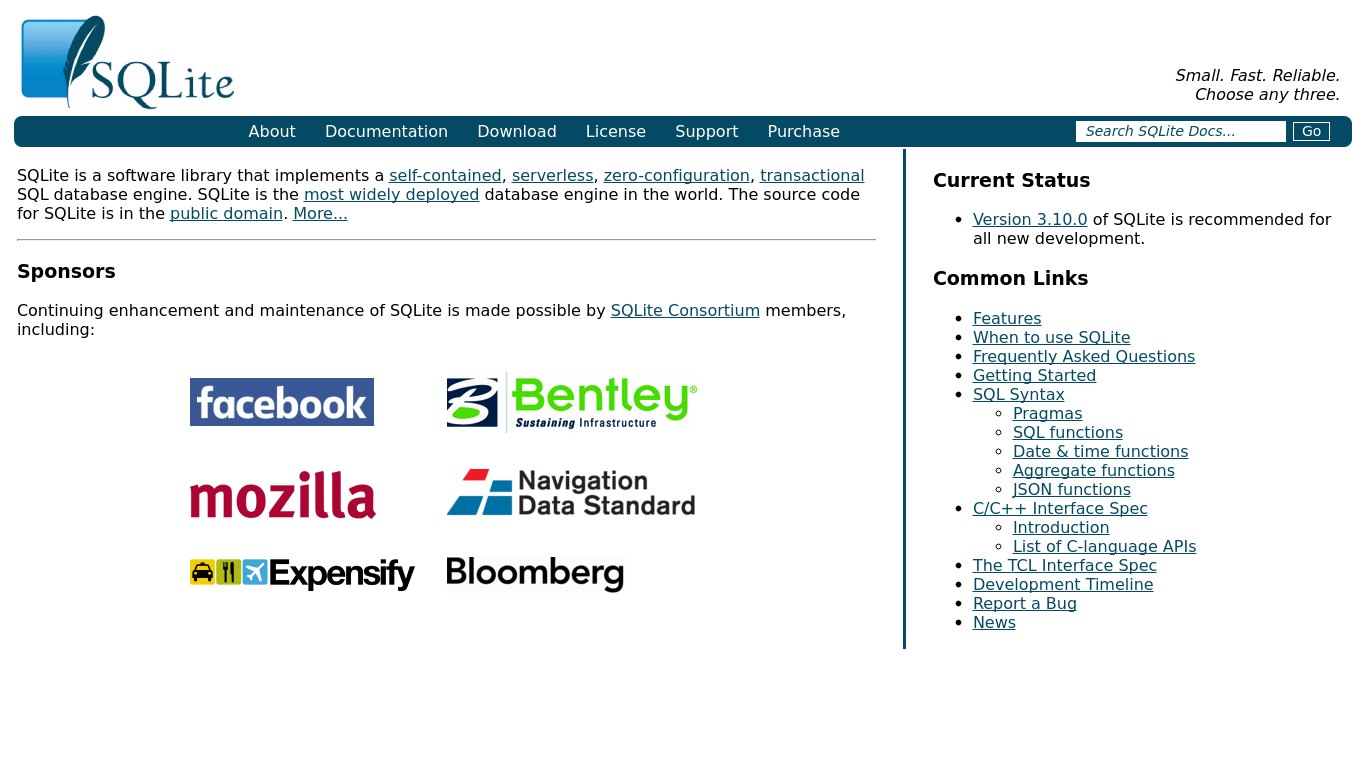The screenshot showcases a detailed view of the SOL Lite website, offering a comprehensive overview of its layout and content. At the top, the website features a clean, white banner adorned with the SQ Lite logo, which is a small white and blue square with a feather beside it. The logo is followed by the text "SQ Lite," with a capital 'L', and the tagline "Small. Fast. Reliable. Choose any three." is neatly positioned in the upper right corner.

Beneath the banner, there is a navigation bar with links to various sections: About, Documentation, Download, License, Support, and Purchase. A search bar with a 'Go' button is located on the far right of the navigation bar.

The main content of the page introduces SOL Lite, describing it as a self-contained, serverless, zero-configuration, transactional SQL database engine. It is touted as the most widely deployed database engine globally. Below this description, the page highlights its notable sponsors, including Facebook, Bentley, Mozilla, Navigation Data Standard, Expensify, and Bloomberg.

On the right side of the page, there is a section titled "Possibilities," featuring links to important resources such as Current Status, Features, When to Use It, FAQs, Getting Started, and Syntax. Each link is clickable, offering users easy access to more detailed information about SOL Lite's functionalities and usage.